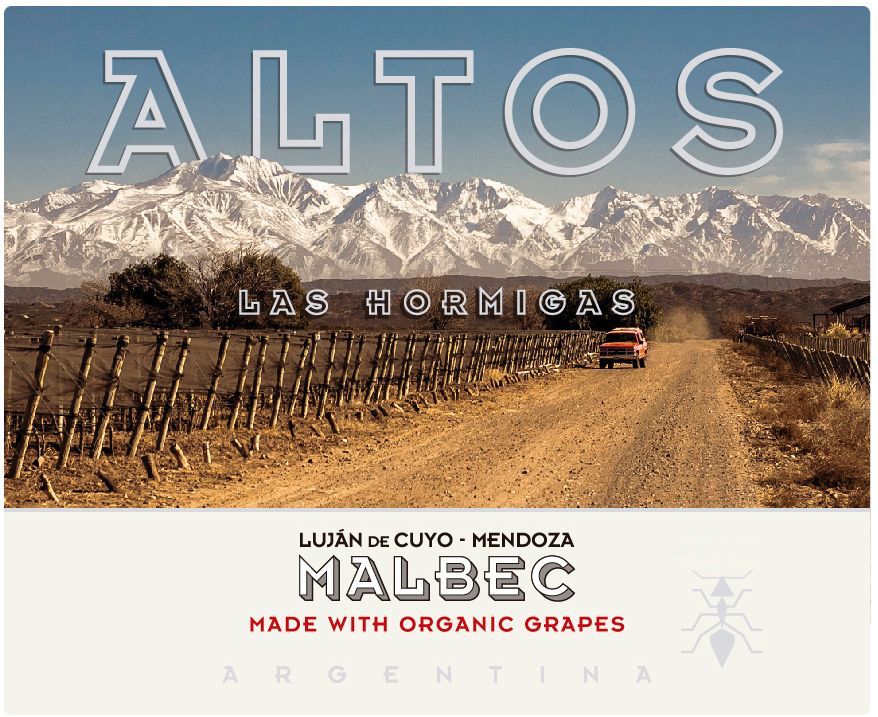The image is an outdoor promotional poster featuring a large rectangular photograph about 5 to 6 inches wide and 3 inches high, depicting a desert landscape during the daytime. In the center of the scene, an old red pickup truck drives towards the viewer on a brown dirt road that stretches diagonally from the right to the left of the picture. The left-hand side of the road is lined with tall wooden posts connected by wire, forming a fence, while on the right side, a dilapidated wooden fence leans precariously. The foreground is dotted with sagebrush, indicative of the arid setting.

In the background, there is a dramatic range of tall, snow-capped mountains beneath a clear blue sky. The text "Altos" is prominently displayed in a light blue, transparent all-caps font across the sky. Below, in smaller white text, it reads "Las Hormigas."

Beneath the photograph, there's a footer with a light gray background, featuring more text. In black print, it says "Lujan de Cuyo," with an asterisk above the "A" in "Lujan," followed by "Mendoza." Below this, "Malbec" is printed in gray 3D lettering, and in red print, it declares "Made with Organic Grapes." Lastly, "Argentina" is written in widely spaced, light gray letters. To the right of this text, there's a small illustration of an ant.